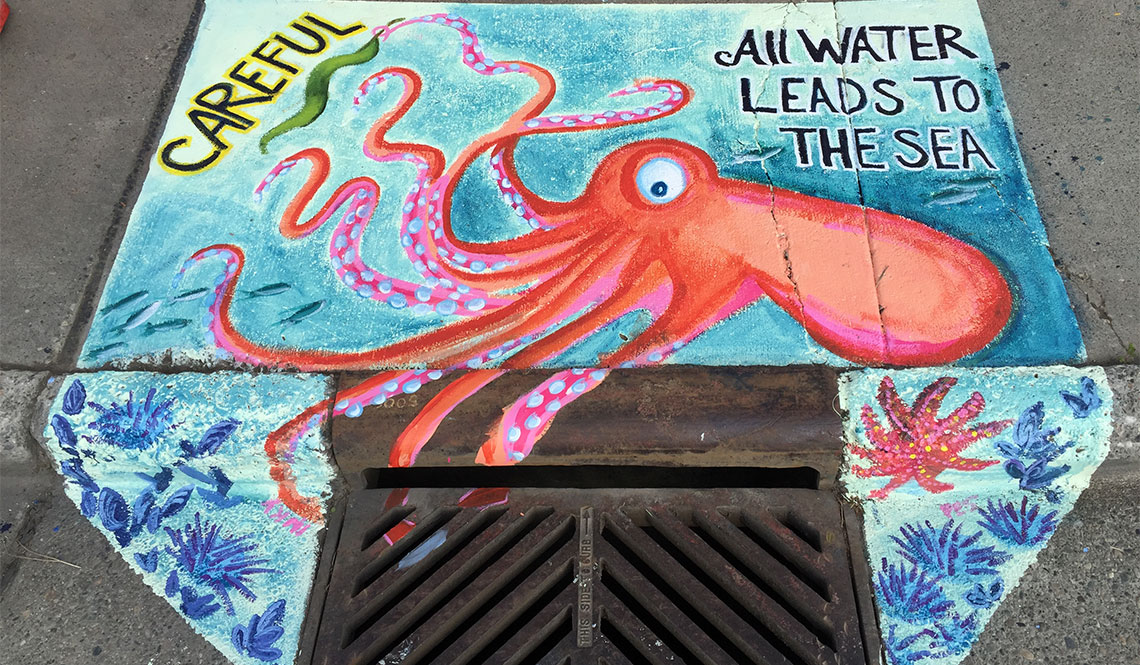The photograph captures a vibrant piece of street art on a concrete sidewalk adjacent to a rusted and black rain gutter. The artwork, executed in chalk, features a pinkish-red octopus with its large, white eye gazing toward the camera. The octopus dominates the right side of the image, with its tentacles extending to the left and some trailing over the edge of the sidewalk, towards the rain gutter. Above the octopus's head, in black lettering, the text reads "All water leads to the sea." On the top left side of the artwork, one tentacle curves around a green leaf, underlining the word "Careful," highlighted in black letters trimmed with yellow. The rain gutter itself is designed with blue coral and shells on the right, and a red starfish, along with more blue coral, on the left. The overall scene delivers a message of environmental awareness, indicating how water from the streets ultimately flows into the sea, reinforced by the merging of the chalk "water" into the rain gutter.